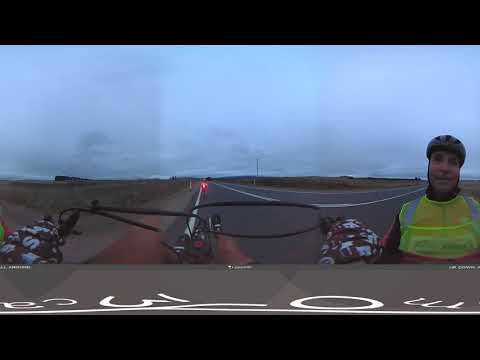The image depicts a somewhat dim and slightly blurry scene of a person cycling down an empty two-lane road during dusk or early evening, under an overcast sky with limited natural light. This scene appears distorted, likely because it’s a 360-degree or panorama image squashed into a flat presentation. The road, made of black asphalt, has white lines on the left, right, and center, indicating traffic divisions, and stretches through flat, almost barren fields with minimal vegetation or trees. The male cyclist, positioned in the bottom right corner, is equipped with a black safety helmet and a reflective yellow-green vest with safety patches. His gloved hands firmly grip the black bicycle handlebars and brake lines. Ahead of him is another cyclist, identified by the red light on their bicycle. The landscape is sparse, and the setting suggests a feeling of isolation, further emphasized by the faint outline of electrical wires in the background. The image also features black bars on the top and bottom, suggesting it might be a still from a video recording.